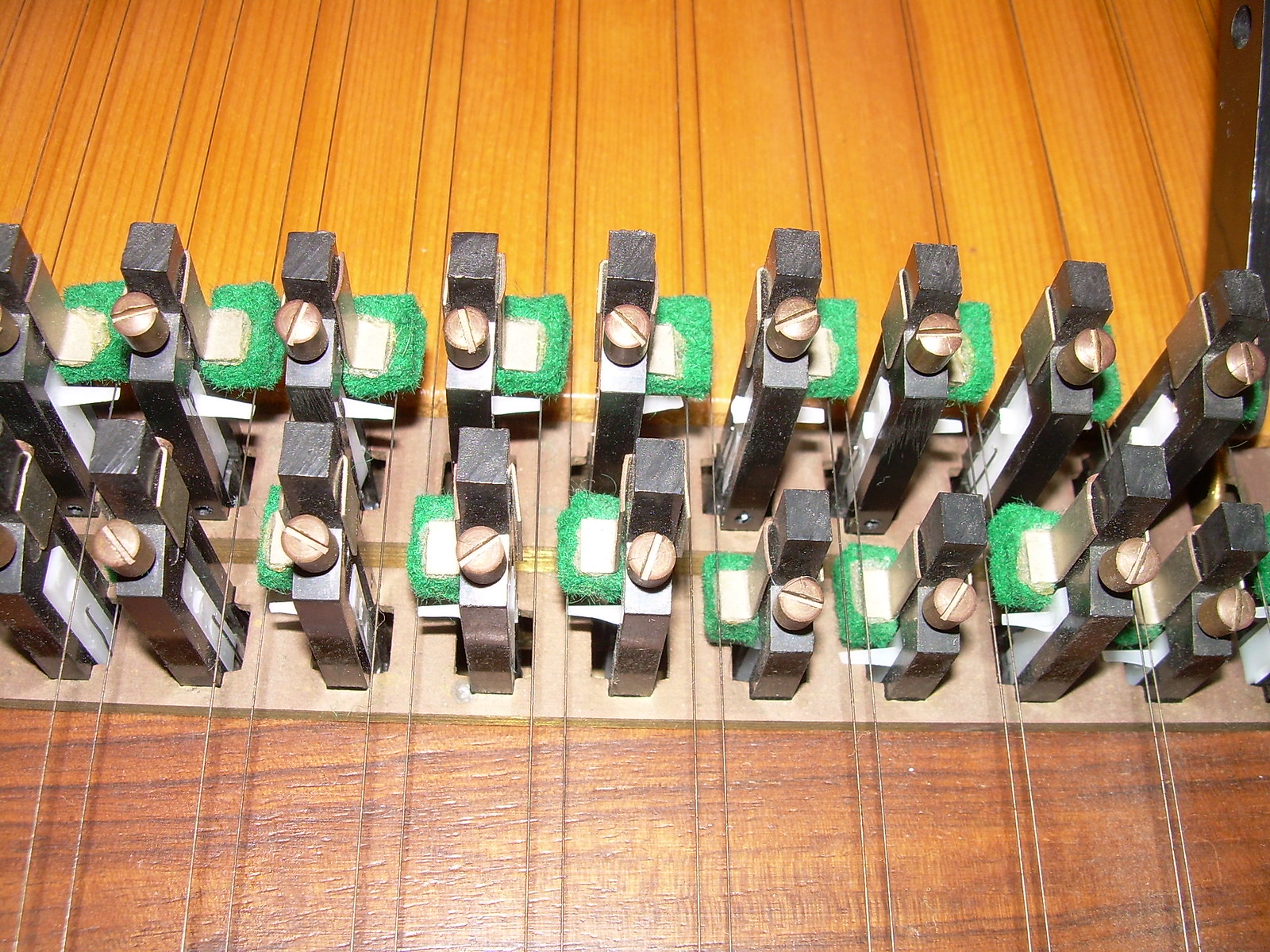This photograph showcases a mechanical apparatus likely associated with a stringed musical instrument, possibly in the family of harpsichords or auto harps. The scene captures two rows of black components of varying heights, each featuring a brass-colored Phillips head screw on top. These components are positioned on a brown, wood-paneled background, with the panels running vertically and a narrow, lighter wooden board positioned horizontally across them.

Each black component has a piece of green and white material, resembling styrofoam, attached to its side. The lower row of components has the green and white pieces on the left, while the upper row has them on the right. There are metal brackets attached to the green and white pieces, which lie against the faces of the black components. Throughout the image, pairs of strings extend from the components, suggesting their role in tuning or holding the strings of the instrument. The presence of both light and dark wood adds to the intricate and mechanical aesthetic, further hinting at the complexity and precision required in the instrument's construction.